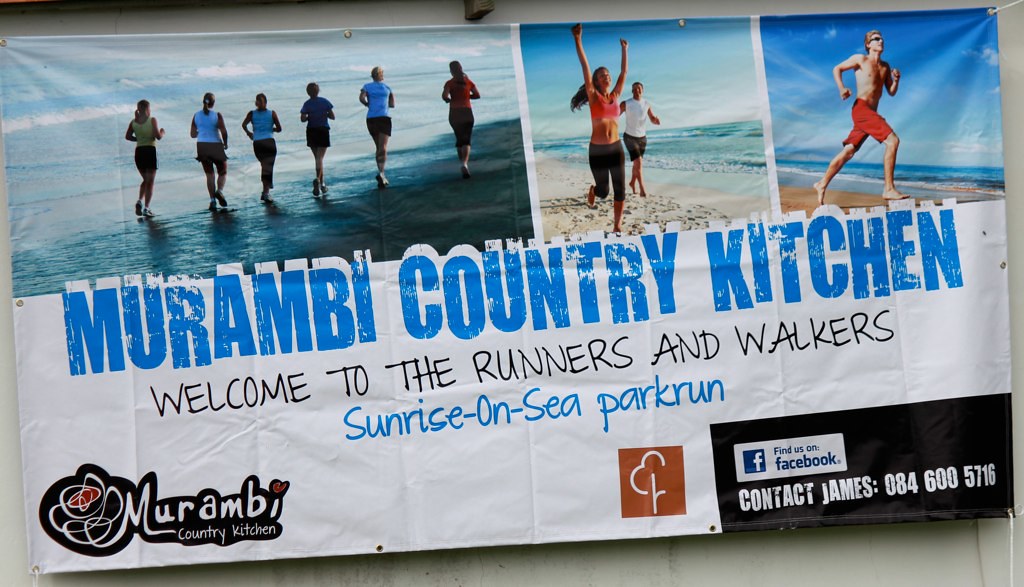This landscape-oriented photograph captures a detailed banner displayed against a white wall, likely made of tarp material with visible grommets and strings in the corners. The banner features a white background with three colorful, horizontally-aligned photographs across the top. 

The far left photograph shows six women running away from the camera on a beach, emphasizing their backs against the scenic backdrop. The central photograph captures a man and woman also running on the beach, this time towards the camera; the woman is leading with her arms raised joyfully, and the water is visible to the right. The third photograph on the right depicts a solitary man in red shorts and sunglasses running on the beach, with the distant water and sandy shore setting the scene.

Across the main center of the banner, large blue uppercase letters spell out "Morambi Country Kitchen," prominently overlaying parts of the photographs above. Below this title, black text warmly welcomes visitors with the phrase, "Welcome to the Runners and Walkers," followed by blue text announcing the "Sunrise on Sea Park Run."

The bottom left corner of the banner displays the distinctive Morambi Country Kitchen logo, a black-and-white design with a touch of red. Towards the center right, there is an orange box featuring what appears to be a partial tree image. Rounding off the bottom right corner is a black rectangle containing the contact information, "Contact James 084 600 5716," and the Facebook logo, inviting viewers to find them on social media.